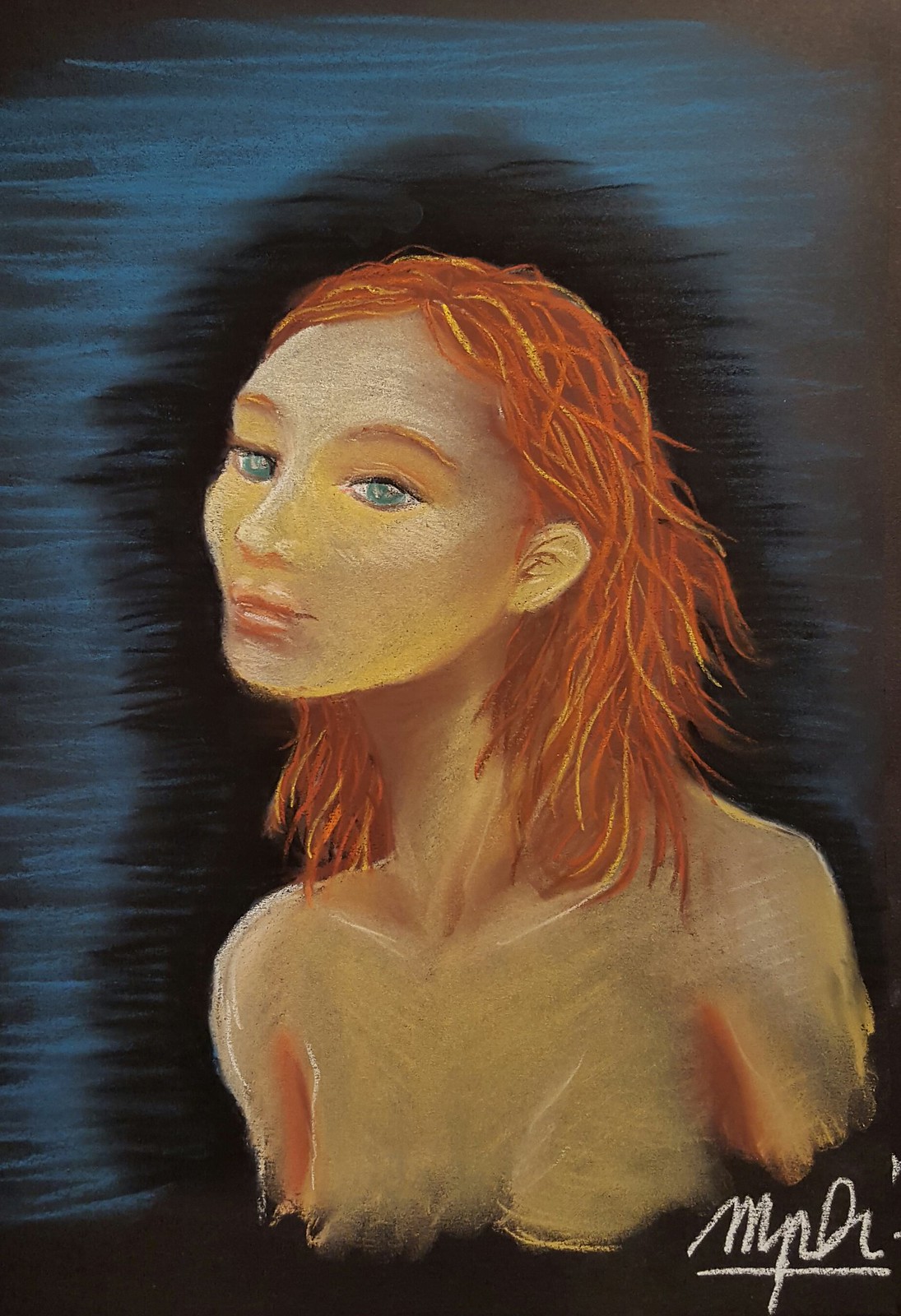A detailed pencil and chalk sketch features a young redheaded woman with striking greenish-teal eyes. Her hair, adorned with blonde and yellow highlights, cascades down to her shoulders, resembling spaghetti noodles. She has pronounced orange eyebrows, and her lips exhibit a gradient from a peach-colored upper lip to a darker, reddish-orange lower lip. The young woman, who appears to be in her early to mid-teens, is partially unclothed, revealing her clavicle, neck, shoulders, and the upper breast area without displaying nudity. The sketch is framed by a black outline with a subsequent blue outline. The background is dark, accentuating the subject. The woman is gazing towards her right. In the bottom right corner of this vertical piece, a partially cut-off signature, presumably the artist’s, is inscribed in white script and underlined, possibly containing the initials MP.